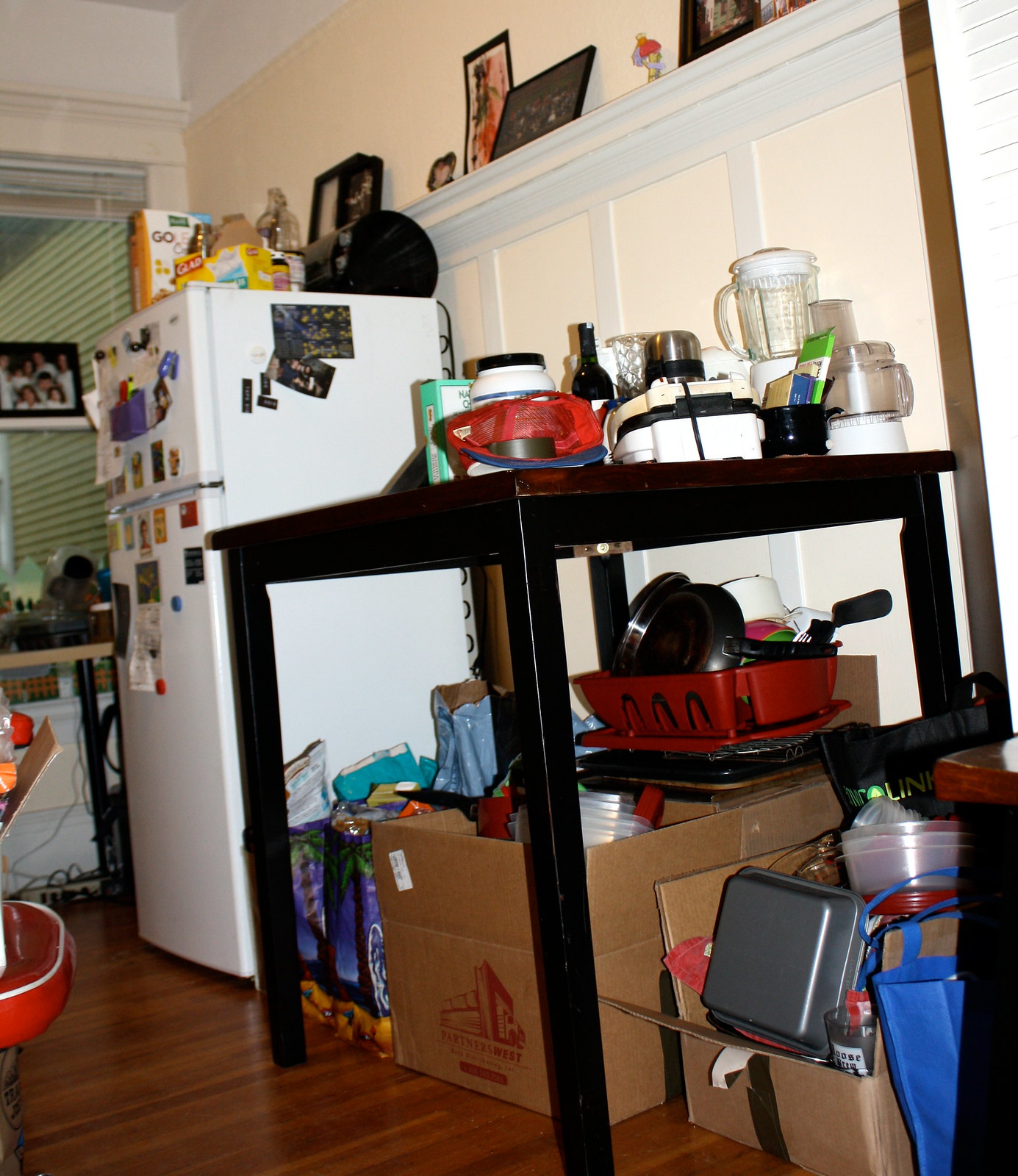This photograph captures a cozy kitchen space in a home. On the far left, a wall-mounted mirror reflects a picture or a mini blind. Next to the mirror stands a white refrigerator adorned with various pictures and items on both its front and visible side. Adjacent to the refrigerator is a tall, black dining room table which extends towards the foreground, laden with kitchen utensils, dish drainers, pots, and pans stored underneath.

On the countertop, a blender, mixer, and various containers including a waffle maker are prominently displayed. The wooden floor is partially visible, adding warmth to the scene. A red object, possibly a decorative item or kitchen gadget, is visible on the left side. An electrical cord runs along the wall behind the refrigerator. Midway up the refrigerator, there's a half-exposed shelf holding unidentified items. Additionally, the top of the refrigerator is cluttered with boxes, cereal, and other miscellaneous objects.